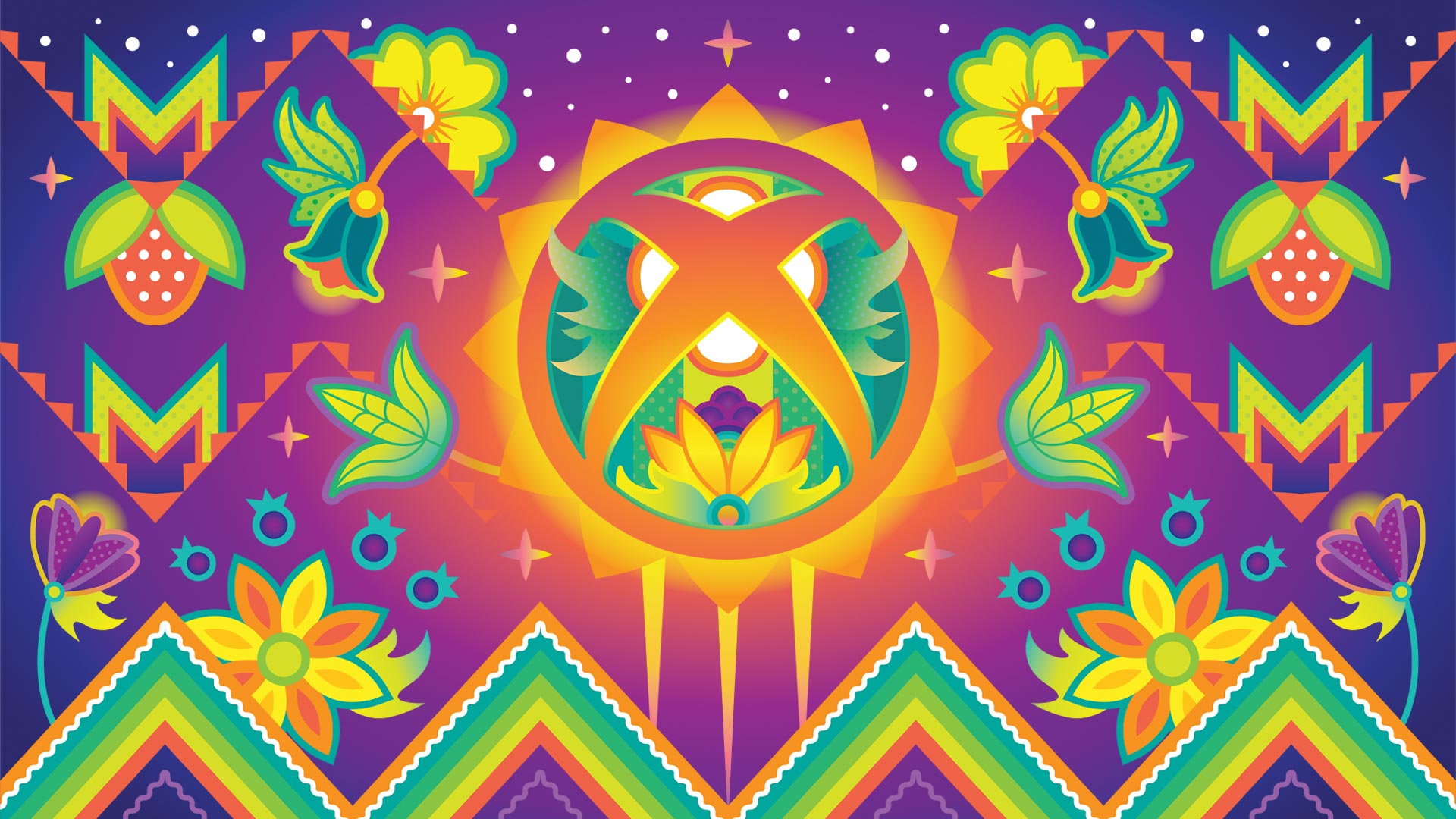The image is a vibrant and detailed artwork featuring a multicolored palette dominated by shades of blue, with significant accents of orange, purple, green, and yellow. The focal point is a central circle resembling a solar sunflower, distinguished by a hexagon across its round center. Surrounding this central motif is a ring of triangles, some of which overlay with a translucent white circle, within which a green sphere and additional triangular shapes can be seen. The design is further adorned with green and yellow 'M' shapes, stars, and white dots, creating a dynamic and clean aesthetic. Scattered throughout are motifs of strawberries, leaves, and bell-shaped plants. The lower portion of the image features an intricate, inverted v-shaped pattern in hues of orange, blue, green, light green, and yellow, contributing to a cohesive yet complex travel poster-like composition.